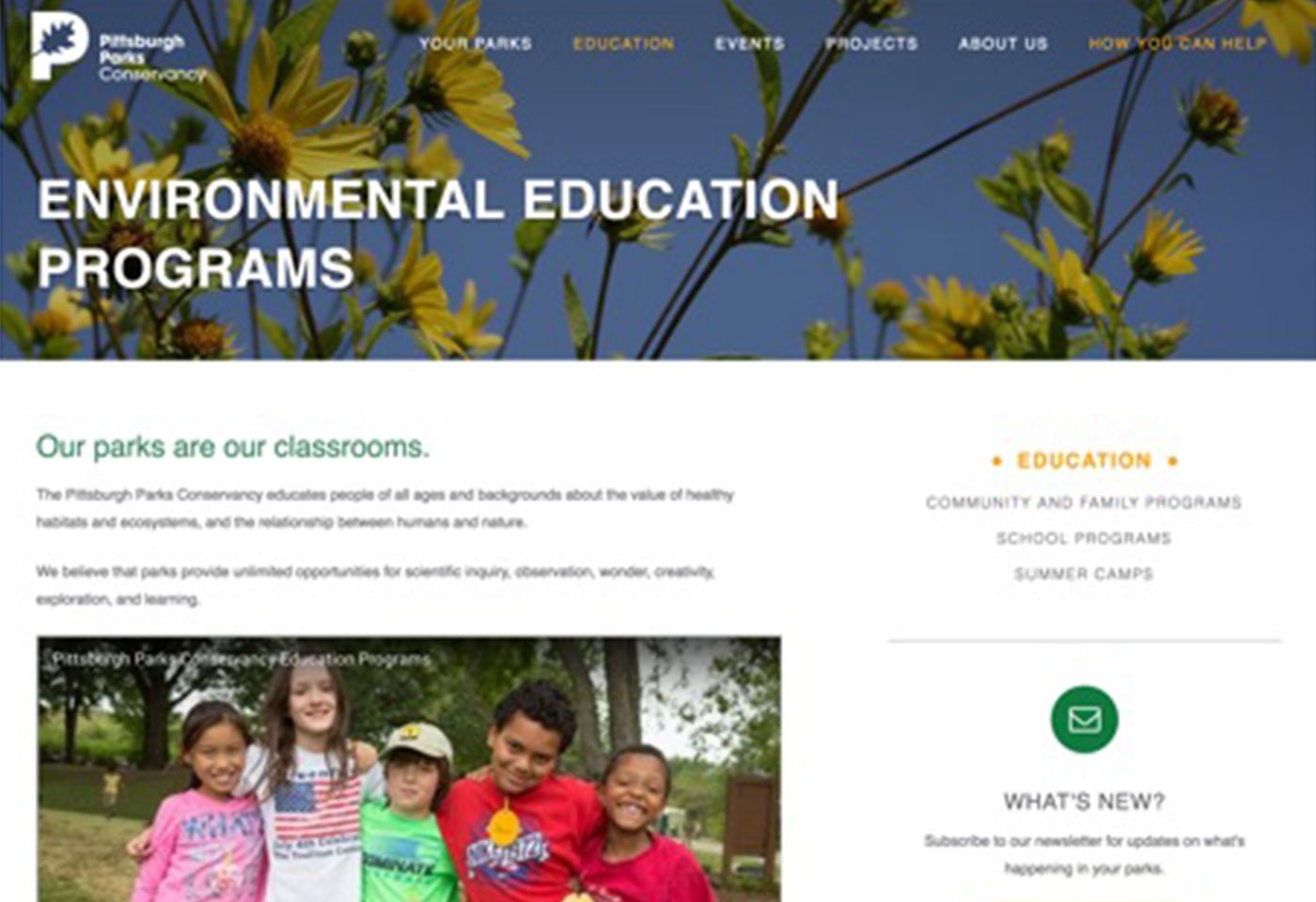This is a detailed descriptive caption for a screenshot from the Pittsburgh Parks Conservancy website.

---

The screenshot showcases the Pittsburgh Parks Conservancy website page dedicated to education, fronted by a blue sky background with dandelions blowing in the wind. The Conservancy's emblem, featuring a white pea with a blue leaf, appears prominently. The top navigation bar includes options for “Your Parks,” “Education,” “Events,” “Projects,” “About Us,” and “How You Can Help.” Beneath the navigation bar, vibrant green text states, “Our parks are our classrooms.” It highlights Pittsburgh Parks Conservancy's mission to educate individuals of all ages about the importance of healthy habitats and ecosystems, and the interconnection between humans and nature. The message emphasizes that parks offer limitless opportunities for scientific inquiry, observation, exploration, creativity, and learning.

Centered on the page is a heartwarming image of five children of diverse ethnic backgrounds – Hispanic, white, and black – hugging each other against a scenic backdrop of trees. On the left side of the photo, a person dressed in pink and lime green attire stands alongside children in white and two red shirts. To the right, a brown wooden park sign, typically found in parks, is visible, with a parking lot situated behind it.

To the right of the image, the word “Education” appears in yellow, followed by sections on “Community and Family Programs,” “School Programs,” and “Summer Camps.” A gray line separates these sections from a green circle containing a white envelope icon. Below, text invites visitors to “Subscribe to our newsletter for updates on what’s happening in your parks” under the "What’s New?" segment.